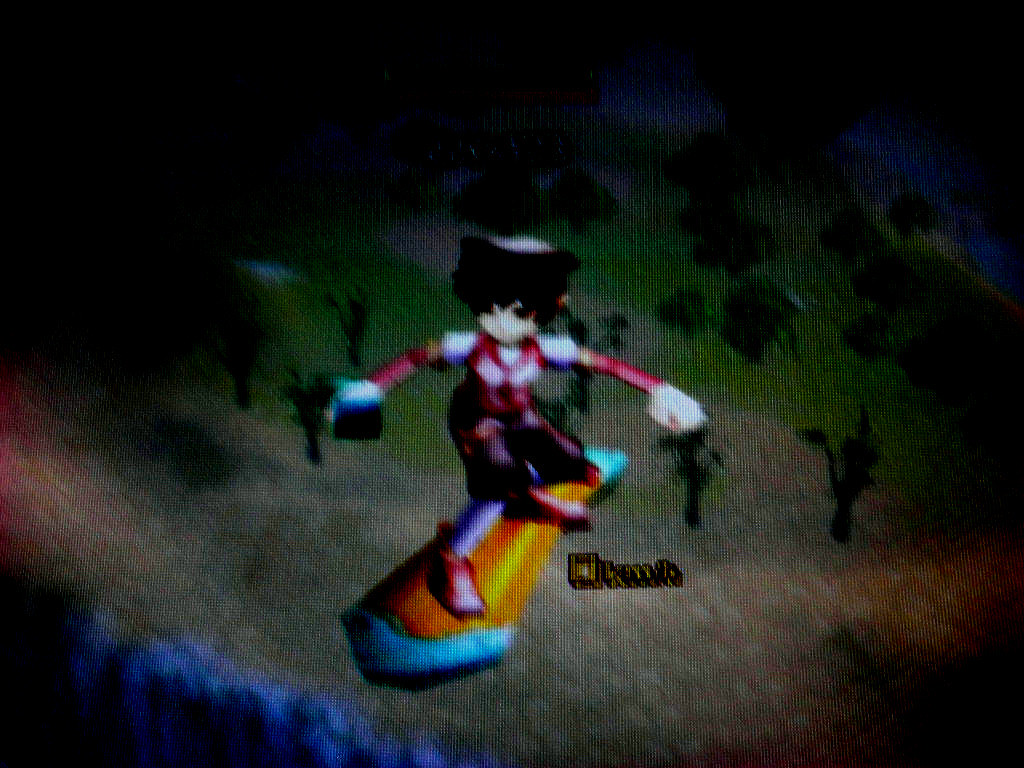A low-quality screenshot from an unidentified video game, featuring a character suspended mid-air atop a surfboard-like device. The device is predominantly yellow with blue accents at the front and back. The character strikes a dynamic pose, feet wide apart and arms outspread, clad in a striking pink vest, matching arm sleeves, and similarly colored shoes. Beneath them, a landscape of winding roads and verdant patches of trees unfolds, with a body of water visible in the background. The scene is unfortunately marred by its dark, grainy quality.